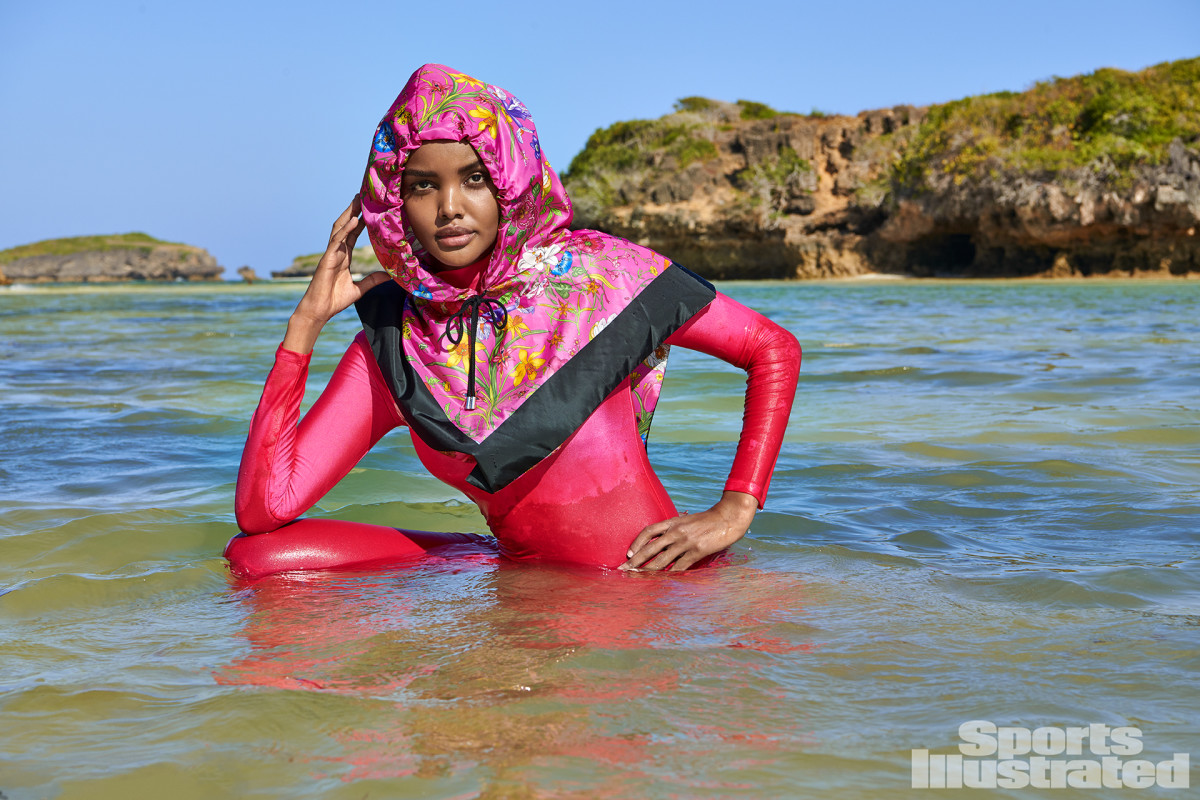In this captivating image for the swimsuit edition of Sports Illustrated, we see the stunning model Halima posing gracefully in the ocean's waters, exuding both elegance and strength. Halima is adorned in a vibrant, pink full-body wetsuit, complemented by a decorative, multicolored headscarf featuring a floral design with a black trim. She is poised in a half-kneeling position, with one knee up, her elbow resting on it while her hand touches the side of her head. The other hand rests confidently on her hip as she gazes directly forward, her expression confident and serene. The water around her shimmers in shades of blue, brown, and green, while the backdrop reveals rocky formations and grassy hills under a clear blue sky, adding a picturesque touch to this iconic and groundbreaking Sports Illustrated cover.